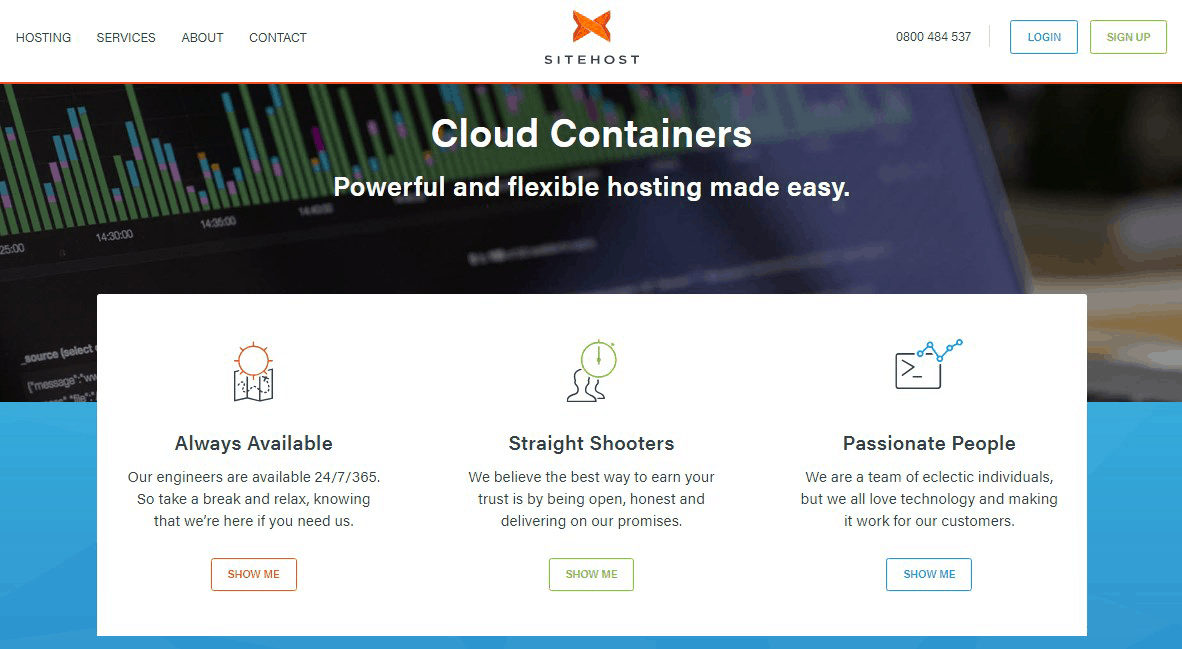The image depicts a webpage from a service provider named "Site Host." The layout is organized and primarily set against a white background.

- **Header Section (Top of the Page):**
  - **Left Side:** Navigation menu with options labeled "Hosting Services," "About," and "Contact."
  - **Center:** An eye-catching orange 'X' graphic, positioned above the "Site Host" logo text.
  - **Right Side:** Contact information "0800-484-537" is displayed, followed by two buttons: a "Login" button with a blue text and blue outline, and a "Sign Up" button with green text and a green outline. Both buttons maintain white backgrounds.

- **Main Content Area:**
  - Central image appears to be a photograph of a computer screen displaying a bar graph.
  - Prominent heading in the upper middle section reads "Cloud Containers, Powerful and Flexible Hosts, Made Easy."

- **Information Section (Below the Main Image):**
  - Features a horizontal white rectangle divided into three segments, each presenting a different service feature:
    - **First Segment (Left):**
      - Title: "Always Available"
      - Description: "Our engineers are available 24/7, 365. So take a break and relax, knowing that we are here if you need us."
      - Button: "Show Me" – white button with a red outline and red text.
    - **Second Segment (Middle):**
      - Title: "Straight Shooters"
      - Description: "We believe the best way to earn your trust is by being open, honest, and delivering on our promises."
      - Button: "Show Me" – white button with a green outline and green text.
    - **Third Segment (Right):**
      - Title: "Passionate People"
      - Description: "We are a team of eclectic individuals, but we all love technology and making it work for our customers."
      - Button: "Show Me" – white button with a blue outline and blue text.

- **Additional Design Detail:**
  - A subtle turquoise strip appears below the white rectangle, adding a touch of color and framing the section effectively.

Overall, the webpage design is clean and straightforward, emphasizing the services and values of Site Host with clear visual and textual elements.